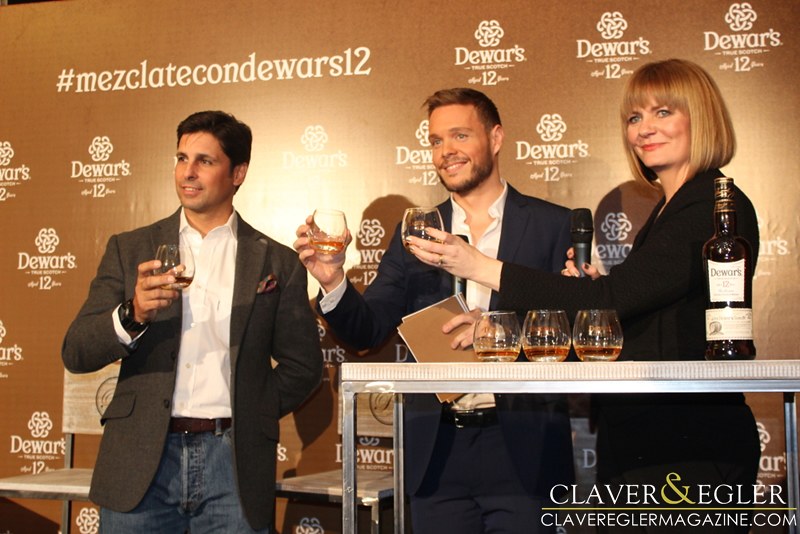The image depicts three individuals standing on a stage, each holding glasses containing a small amount of liquor, presumably Dewar's scotch. The trio consists of two men and one woman. Both men are attired in white button-up shirts paired with suit jackets, while the woman is dressed in a black pantsuit. Notably, the woman, who has blonde hair and appears to be smiling, also holds a microphone in her right hand alongside her glass in the left. 

Adjacent to them, a prominent bottle of Dewar's Scotch is placed on a white-topped table with an aluminum support structure. Additionally, there are three glasses with varying amounts of liquid on this table. The backdrop features a bronze-colored sign with white lettering and Dewar's logos interspersed throughout. This sign also displays the hashtag "Mezcal, Mezclot Conde Wars 12," indicating a thematic or promotional element related to Dewar's. 

Illumination from the right side casts soft shadows, enhancing the warm tones of the scene. In the bottom right corner, there is a watermark reading "Claverine Eggler" and a URL "claverenglandmagazine.com," suggestive of the source or sponsor of the event. A series of interlocking chains and repeated Dewar's branding subtly cover the background, reinforcing the scotch's prominent presence. Two chairs with white padding and aluminum frames are nearby, one positioned next to each man, further emphasizing the staged nature of the setting.